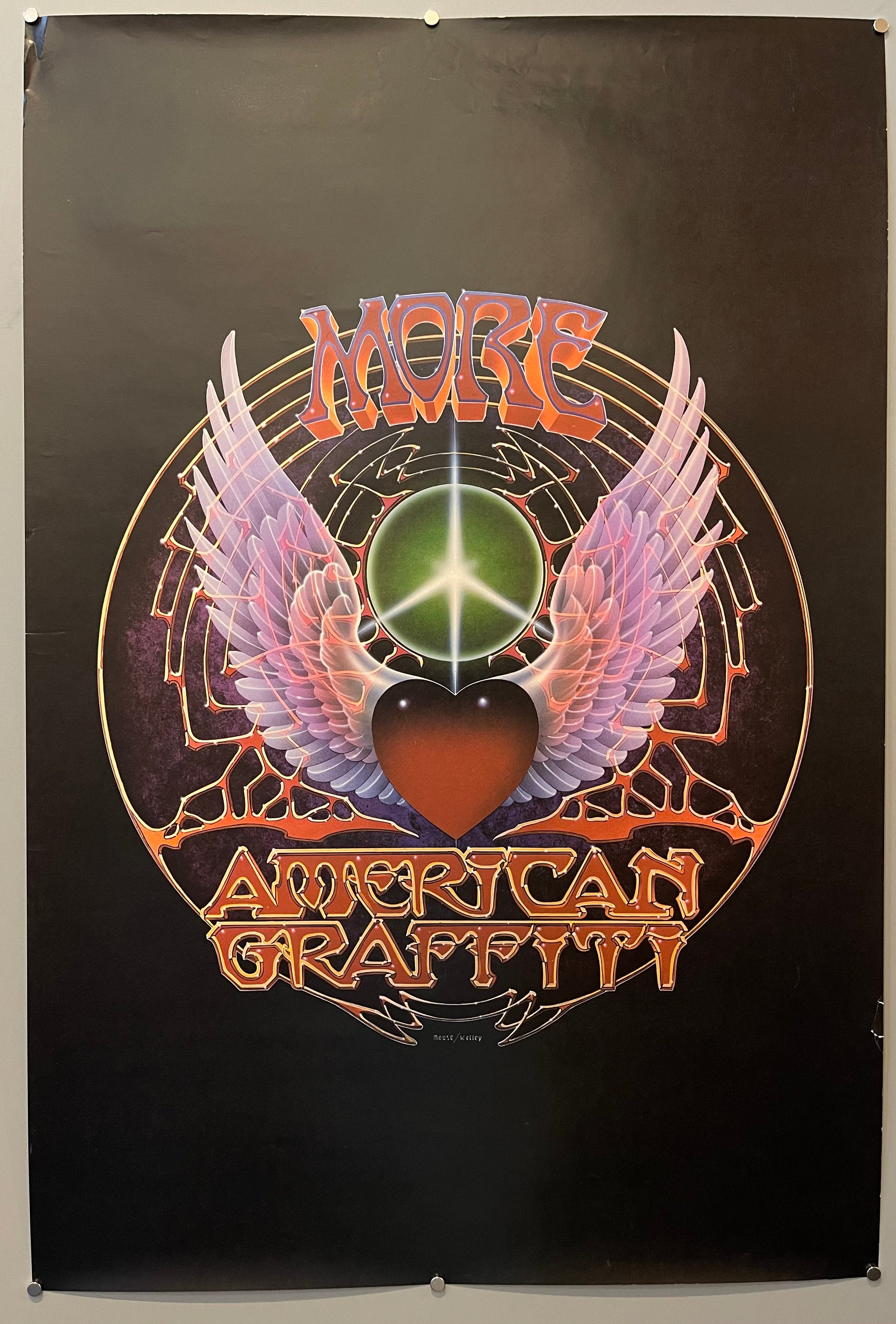This is a poster displayed on a light brown or possibly tan wall, secured with six pins — three along the top and three along the bottom. The poster has a black background and a few wrinkles, especially in the upper left corner, with two small tears near the bottom right pin. The text on the poster prominently reads "More American Graffiti" in stylized letters. "More" is written with raised, textured letters that are primarily red and mixed with purple, highlighted with orange-red effects. "American Graffiti" is rendered in red letters with a gold, gilded outline.

The central emblem on the poster features a large red heart with expansive angel wings. Above the heart, there's a green circle emitting four beams of light in a peace symbol pattern. Extending from the wings is an intricate red and yellow-gold pattern resembling a spiderweb or veins, encircling the heart and adding to the complexity of the design. The emblem and text collectively create a vibrant, eye-catching visual with a mix of graffiti and emblematic elements.